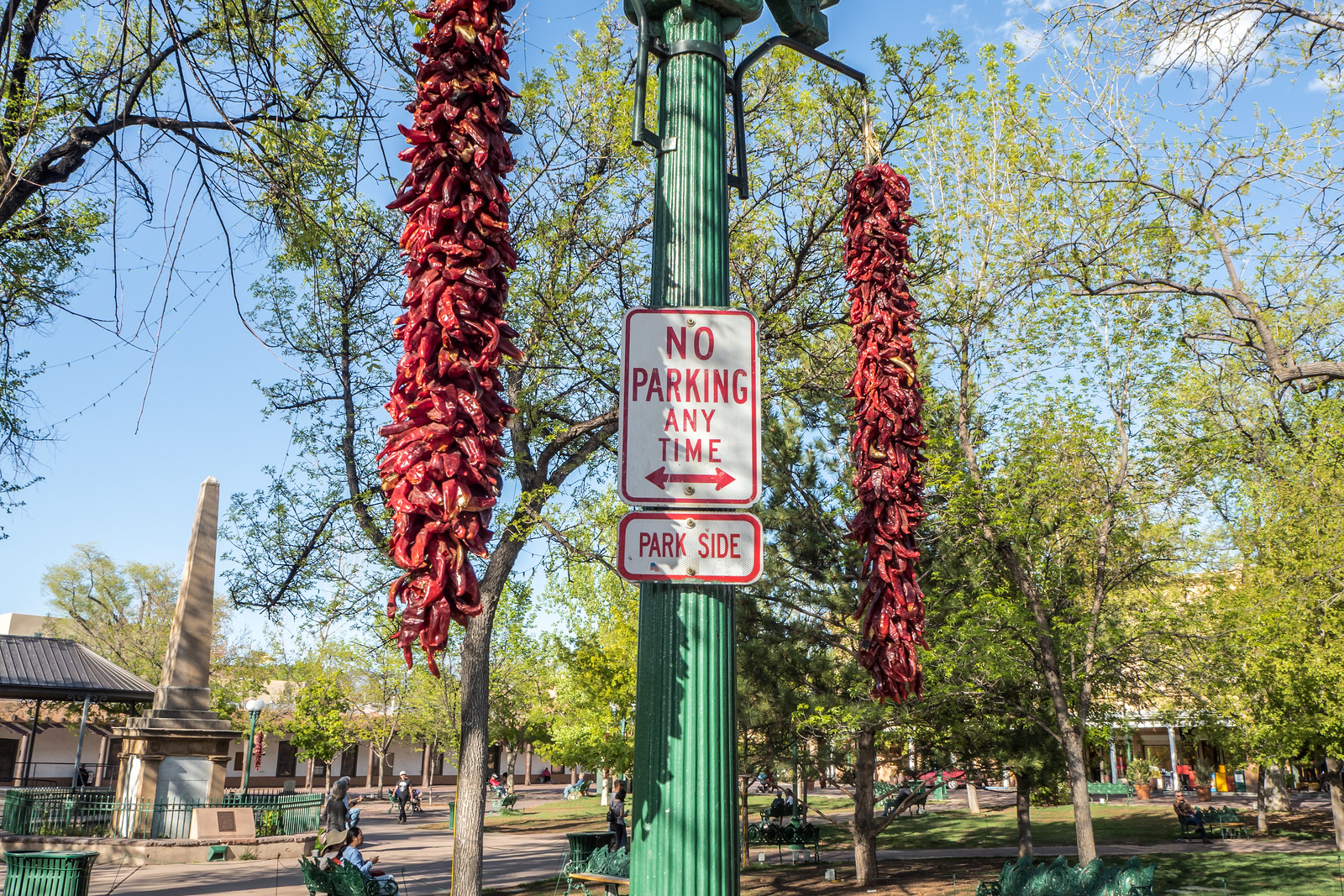In an outdoor park setting, this photograph captures a bright sunny day with a few clouds visible in the top right corner. Central to the image is a tall green metal post adorned with two rectangular white metal signs featuring bold red text and borders. The top sign reads "NO PARKING ANYTIME," flanked by arrows pointing in both directions, while the bottom sign says "PARKSIDE." From both sides of the post, several feet long bunches of red hot peppers hang down, creating a striking visual contrast.

The background reveals a bustling park scene with people sitting on green benches, enjoying the pleasant weather under blue skies. Green trees with brown trunks surround the area, casting dappled shadows on the vibrant green grass below. Several green garbage cans are placed intermittently throughout the park. 

In the distance, a prominently placed gray obelisk monument stands gated off by green metal fencing and features a plaque at its base. The monument is encircled by gray sidewalks that branch out from a central location, defining a layout that draws visitors towards its historic presence. To the right, beyond the trees, partially visible buildings with green rooftops blend into the natural surroundings, completing this serene and picturesque park scene.